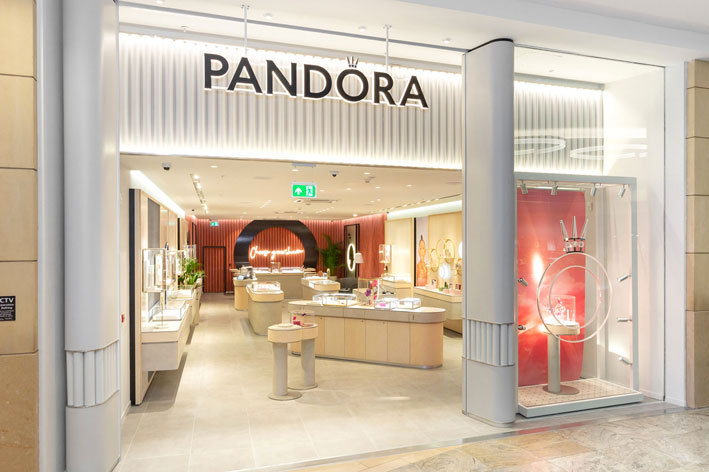The photograph captures the elegant facade of a Pandora store, set within a mall-like environment. Beige stone blocks frame the storefront on either side. The central focus is a large, white-framed window that grants a glimpse into the luxurious interior. Above the entrance, the Pandora logo is prominently displayed in bold black lettering, with the distinctive 'O' styled as a ring with three spikes.

The exterior floor consists of tan tiles, transitioning to light off-white tiles within the store. Inside, the decor exudes sophistication with peach-colored walls and matching beige ceramic tile counters. The interior is well-lit, highlighting glass display cases that showcase an array of jewelry.

Two large white columns mark the entrance, and various standalone displays and benches are strategically placed to feature the store's offerings. The back wall, a striking reddish-orange, hosts a partially obscured neon-lit sign with a central black circle. In the back right corner, a plant adds a touch of greenery to the otherwise polished setting. Every element of the store is designed to illuminate the products, creating a light, airy, and luxurious shopping atmosphere.